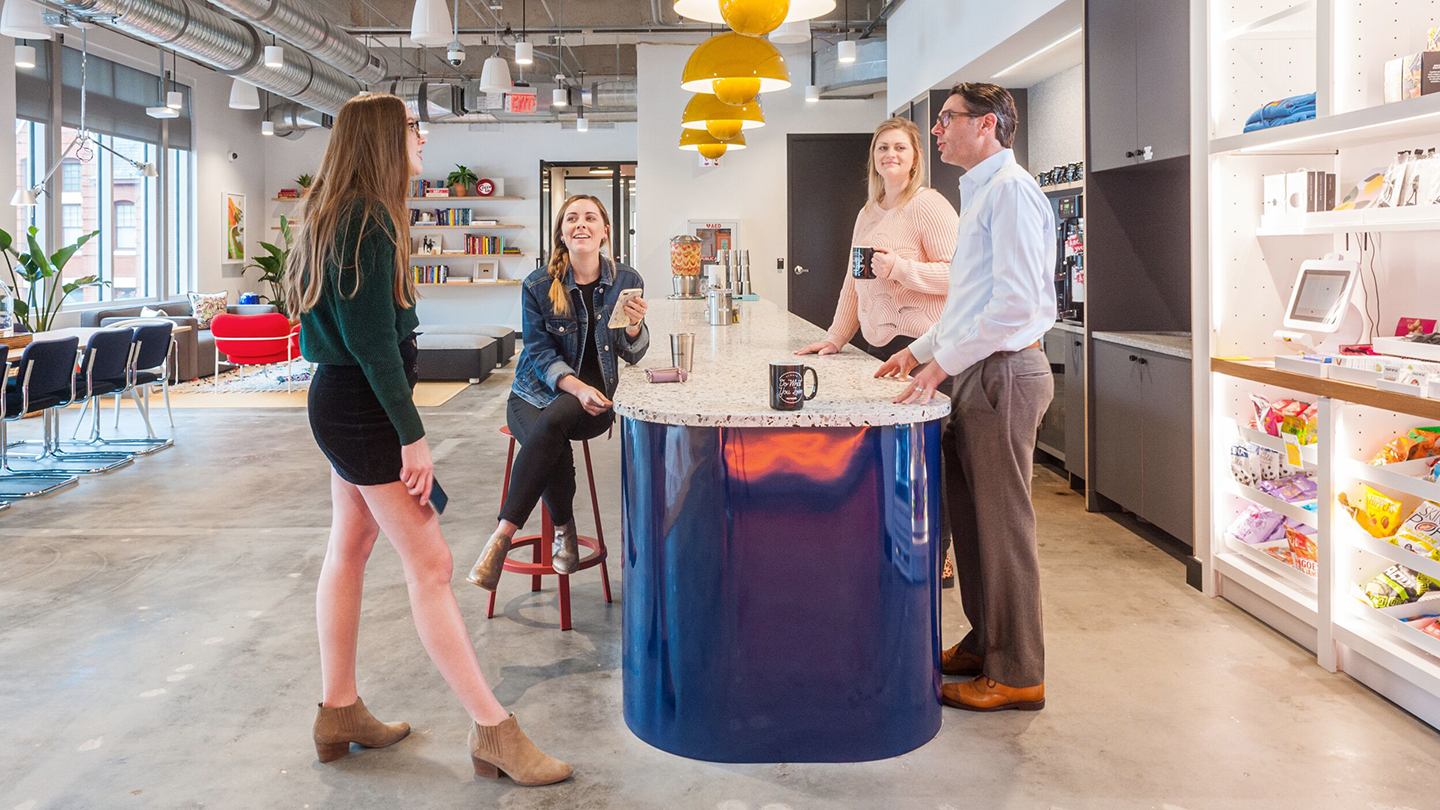The image captures a modern kitchen environment, seemingly within a store or a large meeting room used for breaks. The focal point is a sleek blue island with an extremely shiny, white and black speckled marble countertop, adorned with mugs, tumblers, and various canisters filled with candies and treats. Four adults are engaged in a lively conversation: two younger girls and an older woman in a denim overcoat with black pants, along with an older man. Two of the individuals are wearing glasses. The woman closest to the camera is either standing or sitting on a stool, holding a cup, while another woman has a drink in front of her and is holding a cellphone. The man stands with his hands on the counter. The backdrop features shelves lined with goods, a possible cash register screen, bookshelves, housing plants, and decorative tchotchkes. The space is brightly lit with yellow overhead lights and open ceiling ducts, giving it a warm and inviting atmosphere. Everyone appears to be smiling and engaged, enhancing the casual and friendly setting.